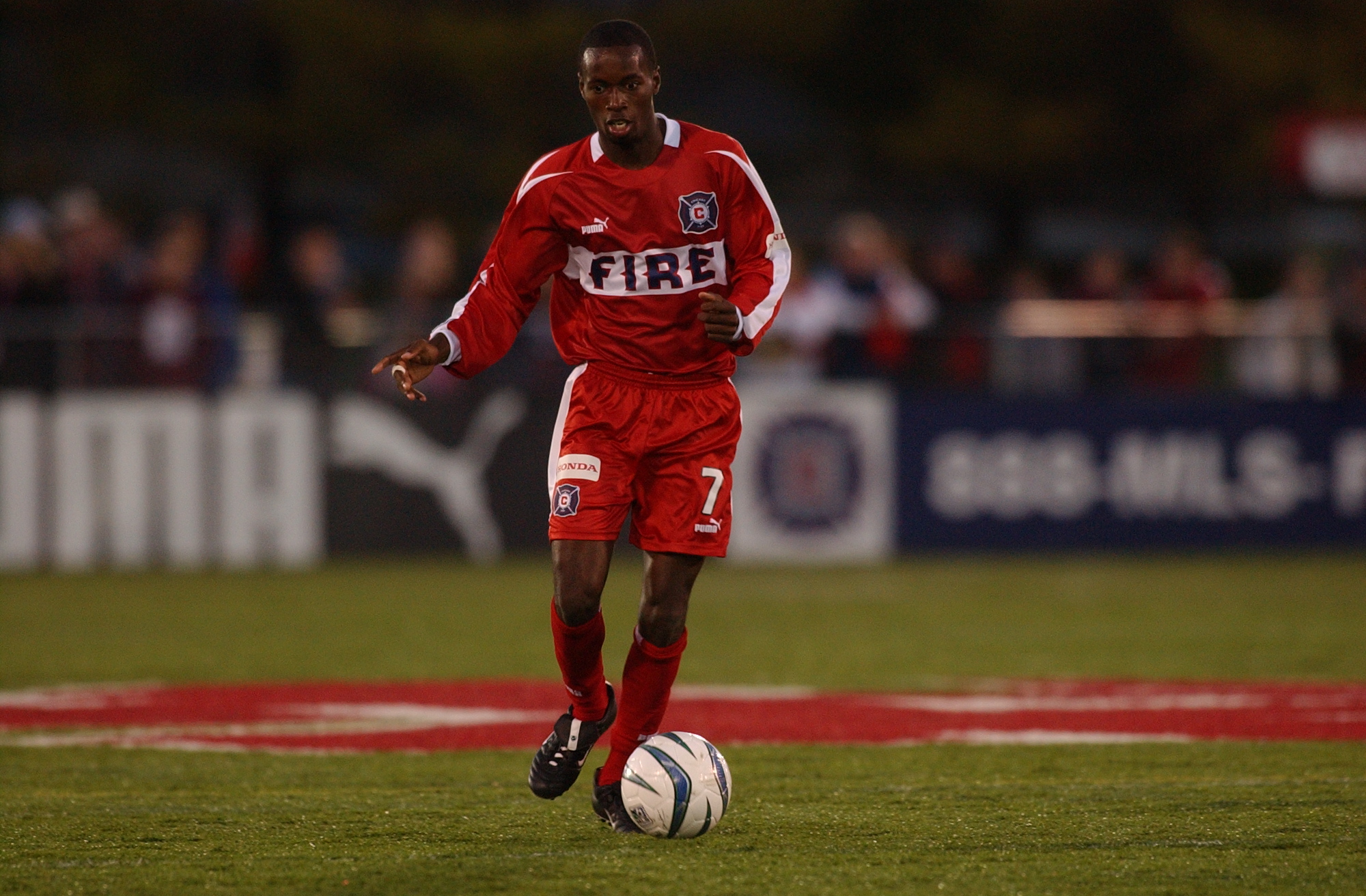In the photo, a professional soccer player is intensely focused as he prepares to kick a black and white striped soccer ball on a green field. He is dressed in a striking red long-sleeved jersey featuring distinct white stripes running from his shoulders to his wrists. Prominently displayed in the center of the jersey, against a white background, is the team name "FIRE" in black lettering, with an emblem of a "C" inside a blue hexagon above the "E". On his left chest lies the Puma logo, and his red shorts, also adorned with white stripes on the sides, display a white "Honda" sticker on one thigh and the number "7" along with another Puma logo on the other thigh. Completing his attire are red socks and black shoes. Amid his determined expression, his right foot slightly off the ground and left foot anchored, the player points with his right hand, possibly signaling to a teammate. The backdrop reveals a blurred crowd of spectators behind a wall lined with advertisements, including a prominent Puma banner, adding to the dynamic atmosphere of the scene.